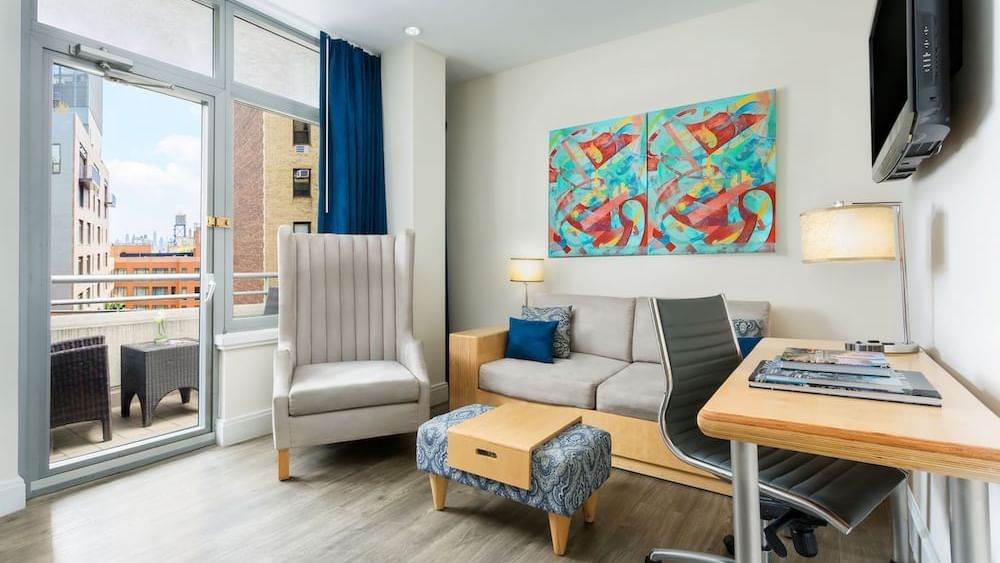The image depicts a brightly lit, modern apartment living room, situated on an upper floor, as evidenced by the cityscape visible through the clear balcony door on the left. The room features white walls and a darkish grayish wooden floor. Dominating the seating area, there is a gray sofa with a wooden frame, adorned with light gray cushions. In front of the sofa, a blue-patterned ottoman serves as a footstool and a convenient drink tray holder. A colorful abstract painting in yellow, blue, and red hues hangs on the wall above the sofa.

Adjacent to the sofa, a velvety light gray chair with wooden legs provides additional seating. The living room also includes a wooden desk with a black chair featuring silver elements, positioned on the right side of the room. Magazines are scattered atop the desk, which is detailed with metal cylindrical poles. To the right of the desk, a sleek black television is mounted on the wall.

Two lamps, one located on the far right and one near the sofa's middle area, cast a warm glow throughout the room. The balcony, visible on the far left through glass doors with blue curtains pulled aside, houses black straw patio furniture—a chair and a small table, possibly holding a plant. The room's vibrant and functional decor is completed by the locked balcony door, which features a deadbolt for security.